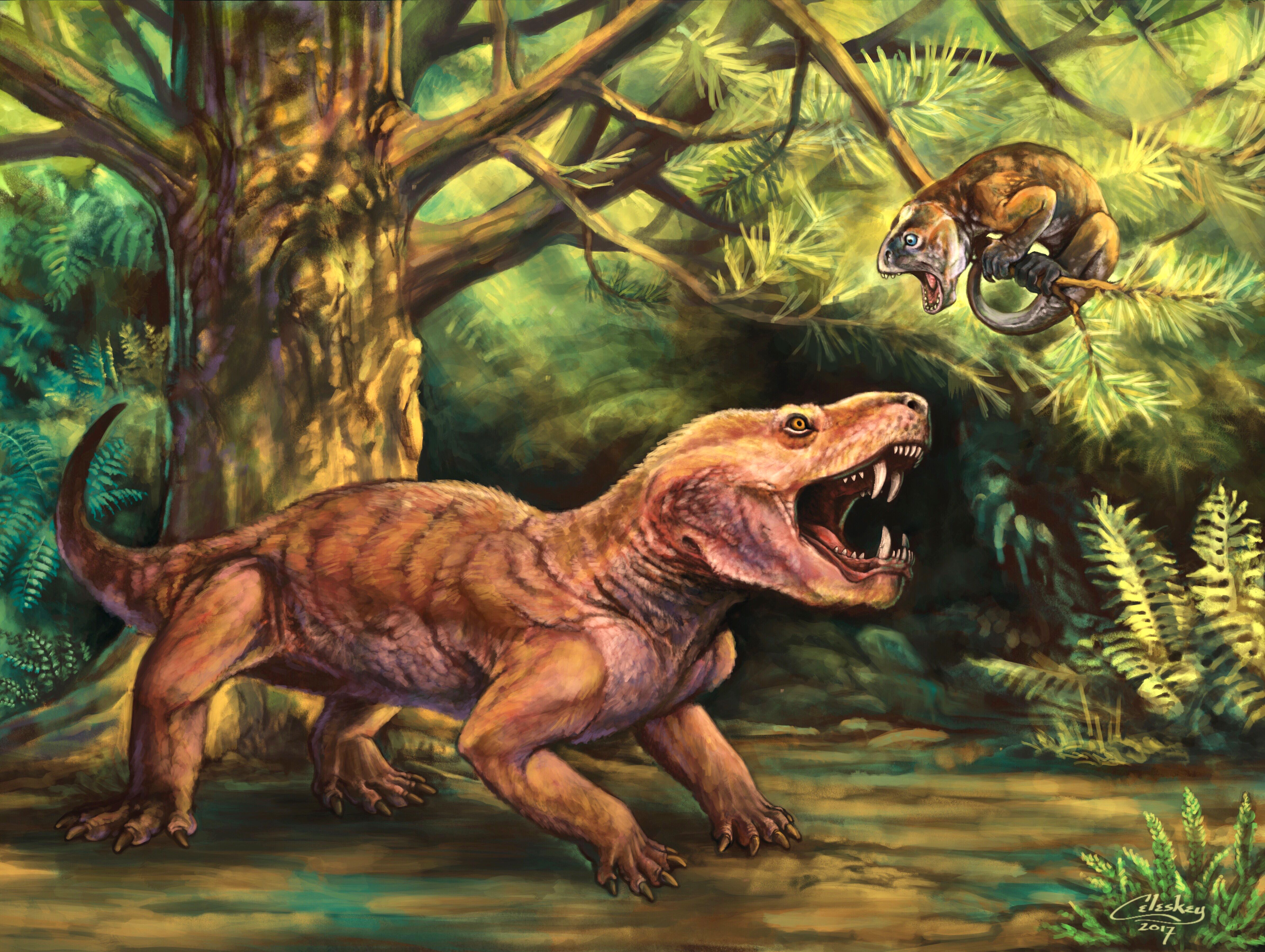In this detailed digital illustration, we see a dynamic scene set in a dense, forested area filled with varying shades of greenery. Dominating the left side of the image is a large tree with a thick trunk and sprawling branches adorned with leaves. The ground beneath is muddy and brown, scattered with ferns and other plants. 

The primary focus is on two prehistoric creatures locked in an apparent confrontation. The first dinosaur, predominantly red and hefty in build, occupies the lower left corner. It stands on four stout legs, positioned diagonally with its back legs furthest and right legs closest to the viewer. The dinosaur has a broad, curling tail, an oversized head, and a body resembling that of a lion or tiger but with distinct dinosaur features such as a lack of ears. Its mouth is wide open, revealing four prominent, sharp teeth, and it has a single yellow eye visible in its right-side profile.

Perched just above this roaring dinosaur on one of the tree’s branches is a much smaller, brown lizard-like dinosaur, roughly the size of an iguana. Its form is tightly wrapped around the branch, gripping it with both hands and feet. It has a rounded head, blue eye, and an open mouth displaying sharp teeth, seemingly engaged in the standoff. 

The illustration is signed in the lower right corner with the name "Saliski 2017," adding an artist's touch to this vivid portrayal of an ancient, primal scene.